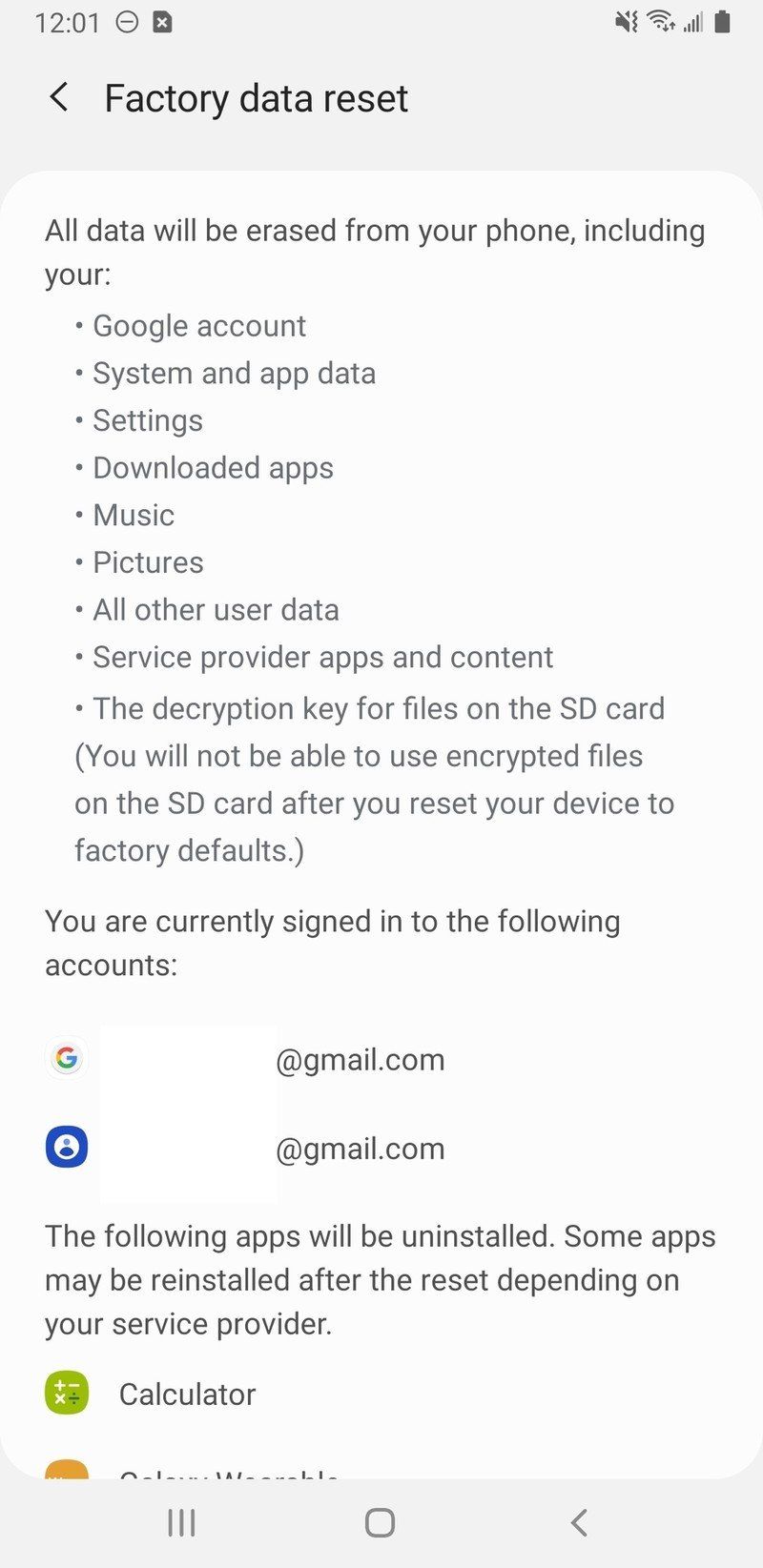This image captures a close-up view of a cell phone screen displaying the "Factory Data Reset" menu. The timestamp on the device indicates it is 12:01. The screen is titled "Factory data reset," and it presents a comprehensive warning about the consequences of proceeding with the reset.

The message informs the user that all data will be erased from the phone, including their Google account, system app data, settings, downloaded apps, music, pictures, and any other user data. It also mentions the removal of service provider apps and content. Importantly, the decryption key for files on the SD card will also be deleted, making encrypted files on the SD card inaccessible after the reset, as noted in the parentheses.

The screen further details the accounts currently signed in to the device, with icons for Google and Samsung, although no specific accounts are visible. The text then states that "The following apps will be uninstalled," with a note that some apps may be reinstalled depending on the service provider. Below this, there is a single calculator icon listed.

The overall scene is one of a clean and straightforward reset interface, providing the user with detailed information about the ramifications of resetting the device to factory settings.